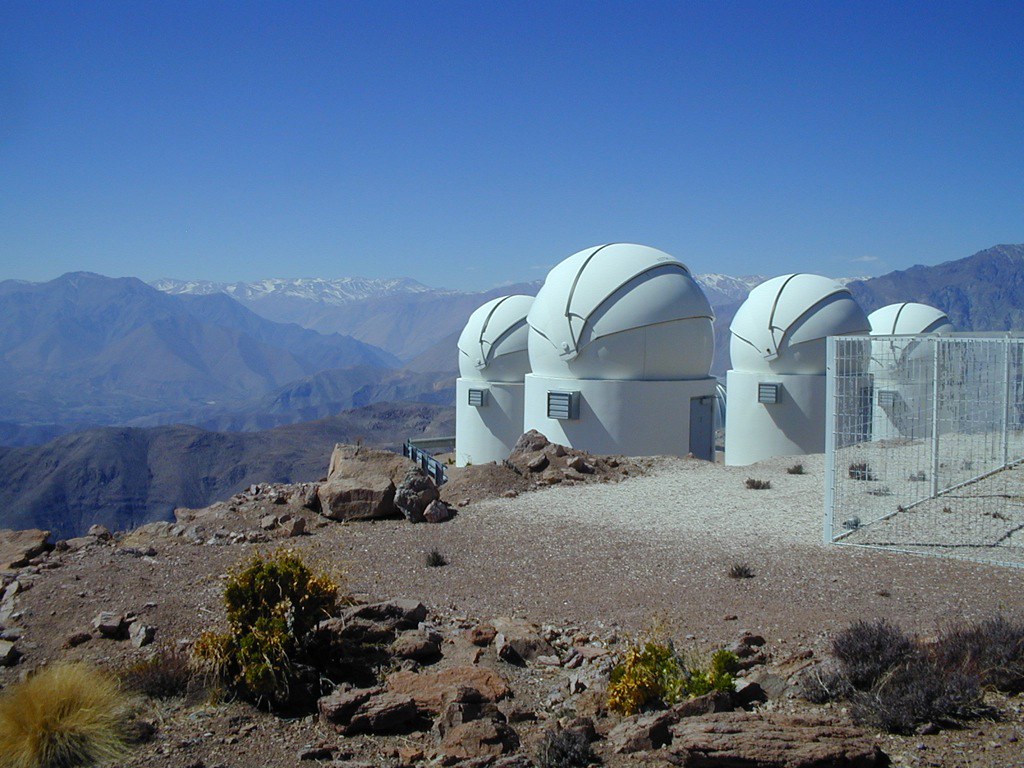The image showcases a high-altitude viewpoint in a desert mountainous terrain under a clear blue sky. Dominating the scene are four circular white observation towers, each featuring a gray vent on their left side and central doors at ground level. These towers are situated on a cliff, overlooking a panoramic vista of rugged brown mountains partially dusted with snow. The area is enclosed by a white wire fence, possibly serving as a safeguarding barrier around a dirt path. The landscape predominantly consists of tan and gray rocks, interspersed with sparse green shrubs, giving a sense of the arid environment. The image hints at a purpose related to either energy conservation or space observation, emphasizing the remote and serene nature of this high-desert location, potentially in a region like California or Nevada.